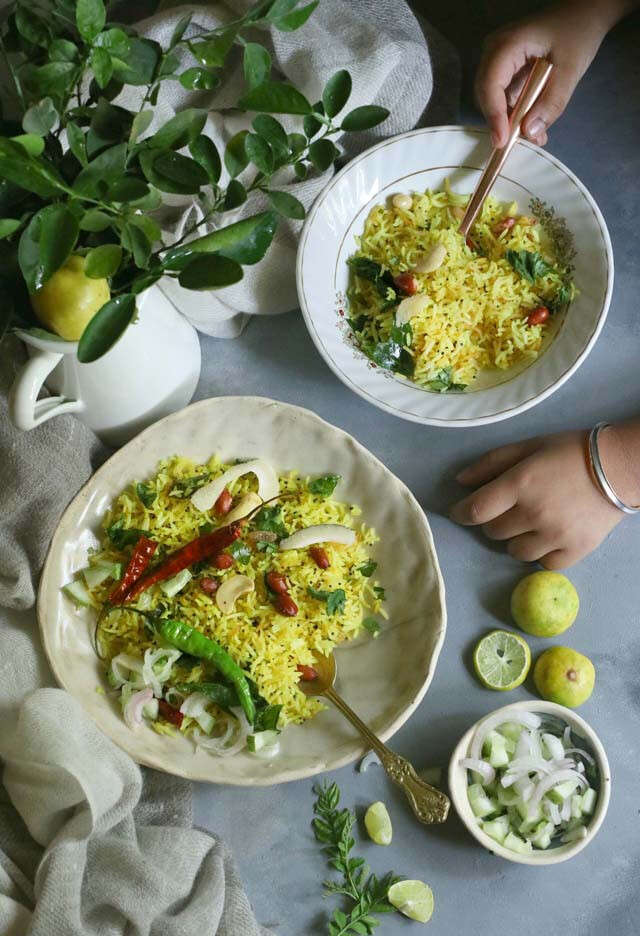The image depicts two Mediterranean-inspired rice dishes garnished with a colorful assortment of vegetables and nuts. Both dishes feature vibrant yellow rice mixed with red and green peppers, cashews, and various green herbs, likely mint or cilantro. The larger bowl, located in the center of the image, has a mix of these ingredients along with some red beans and pieces of greenery. Adjacent to it, a smaller bowl also contains the same yellow rice and garnishes and is positioned at the lower bottom corner of the frame.

Set against a blue tablecloth, additional elements in the scene include a small bowl of onions and potential cucumbers, yellow lemon slices, and a couple of limes. In the background, there's a plant with a cup beneath it. A pair of Caucasian hands, holding what appears to be copper chopsticks or a spoon, is seen eating rice from the larger bowl.